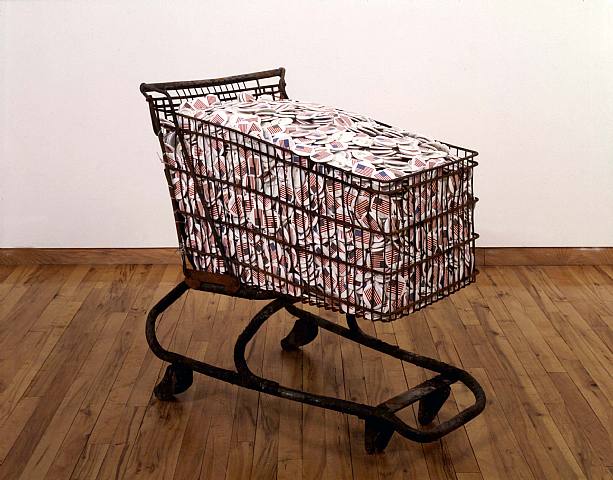This photograph, titled "Collateral" by Hans Hocke, captures a black shopping cart positioned in the middle of an indoor room. The cart, which features a black frame and black wheels, is inclined from the top left-hand corner towards the bottom right-hand corner. It sits on narrow hardwood planks with visible imperfections, adding texture to the scene. The background showcases an off-white, blank wall without any frames or decorations. The focal point of the image is the fully loaded cart, brimming with small, circular stickers or buttons. Each sticker is identical, featuring a graphic of the American flag without any accompanying text.